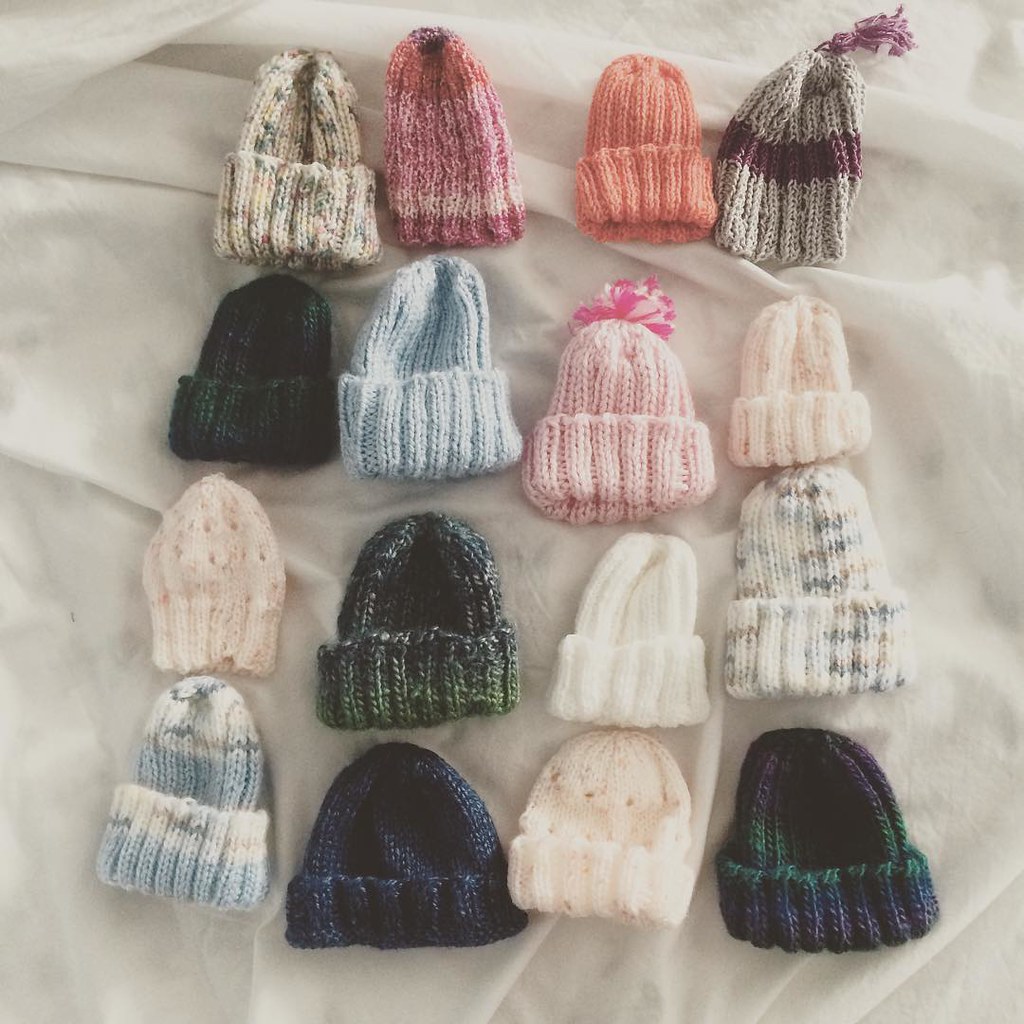This image showcases a neatly arranged collection of 16 handcrafted toboggans and winter caps, ideal for social media or an Etsy advertisement. The caps are meticulously spread out on a white blanket or bed sheet, laid out in four rows of four. Each beanie is unique, made from wool or yarn, featuring a variety of colors and patterns. The top left toboggan is off-white with green speckles, next to it is one with pink shades and a white stripe at the bottom, followed by an orange one that’s partially rolled up, and a mostly white one with a burgundy stripe and a purple tassel. The second row starts with a dark green cap, then a light blue one, a pastel pink with a pink tassel, and a smaller pale pink cap. The subsequent rows exhibit an array of colors, including darker blues and greens. Some of the caps are adorned with pom-poms while others are not, all lying on a cozy blanket, showcasing an appealing and cozy winter accessory collection ready for sale or display.